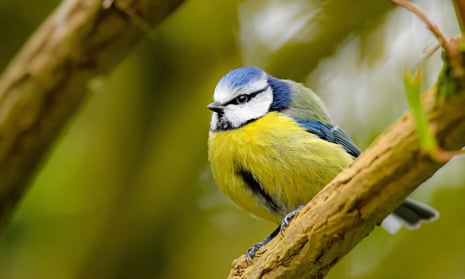This close-up photograph, taken in natural lighting, showcases a small, round, fluffy bird with soft-textured feathers perched slightly to the right of the center on a light yellow branch, which extends diagonally from the bottom center to the middle right side of the image. The bird features a predominantly white face accented with a striking black stripe running from its beak, across its eye, and towards the back of its head. It possesses a black beak, and blue feathers crown its head, transitioning into a collar of blue and a yellow back with hints of yellow-green and blue hues. The underside of the bird is primarily yellow, segmented by a central black stripe. The bird's wings are partially visible, with blue tips extending slightly behind the branch. Its tiny feet grip the branch securely, and a single green-yellow-beige leaf is visible on the right. The background is a soft, out-of-focus blend of green, black, and white, indicating a blurred landscape, perhaps a forest setting, which adds depth to the vibrant subject in focus.